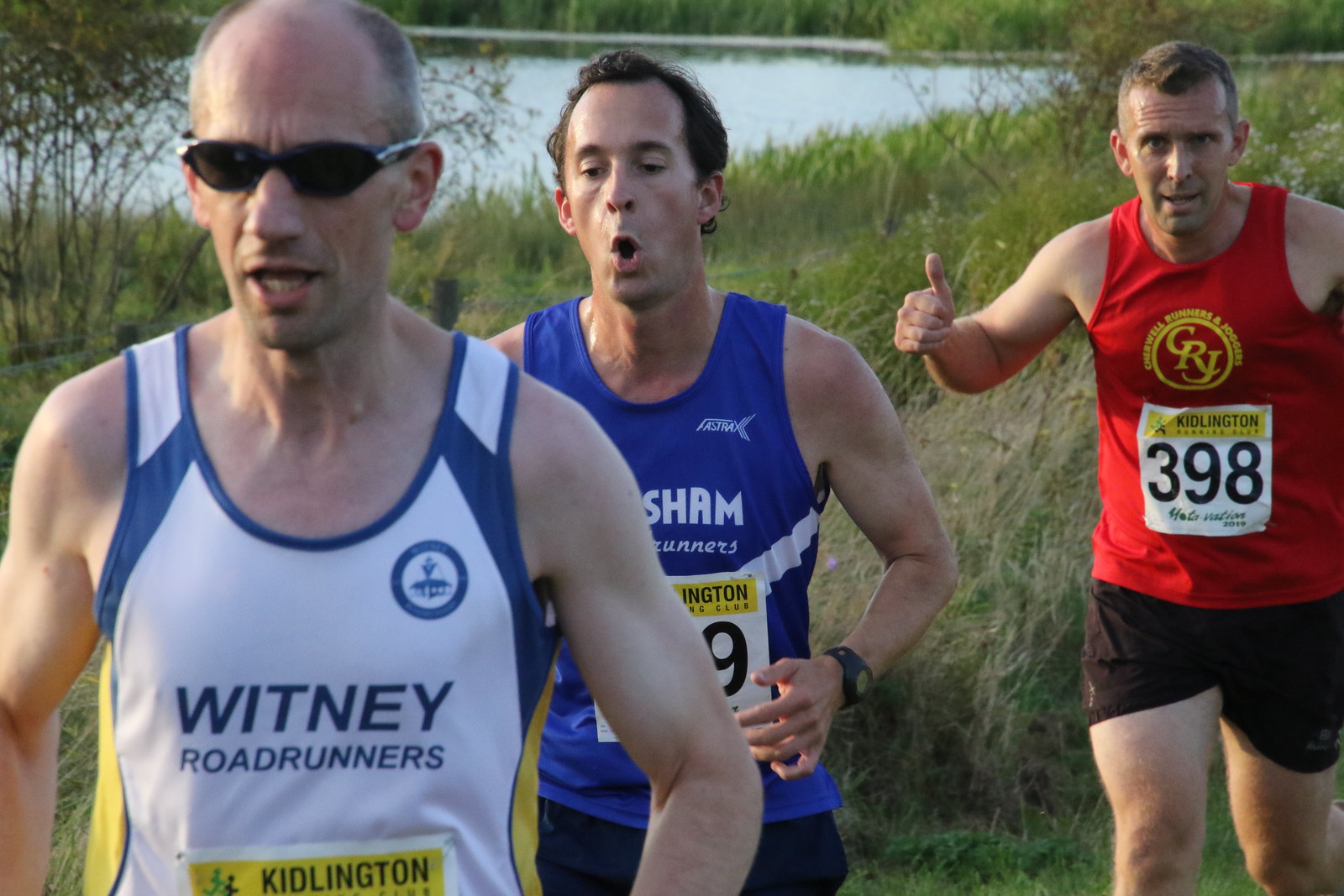This photograph captures three Caucasian men running in what appears to be a marathon or professional jogging event. All three are wearing tank tops and sporting participant numbers, indicating warm weather and competitive context. The scene is set against a backdrop of thick grass and trees, with a large pond or small lake in the distance. 

In the forefront, a middle-aged, bald man with sunglasses is seen. He wears a white tank top that reads "Whitney Roadrunners" and has a tag indicating "Kidlington," though his number is obscured. Behind him to the left, a younger, brown-haired man in a blue tank top is partially visible. Due to his position, the text on his top is not clearly readable. To the right, another middle-aged man with brown hair is captured giving a thumbs up. He is wearing a red tank top with "CRJ" visible and bears the number 398. The scene conveys a sense of camaraderie and competition among the runners.